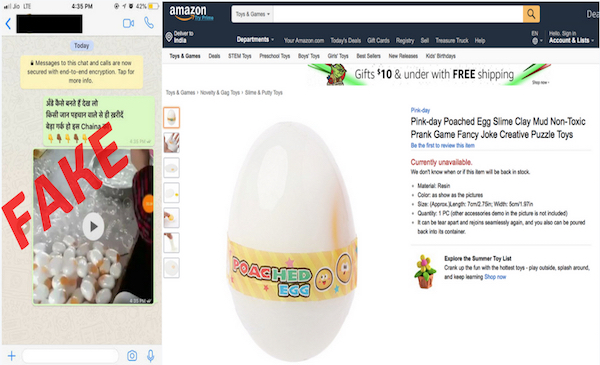On the left side of the image, there appears to be a screenshot from a messaging application, likely WhatsApp. The top-left corner is obscured by a large black rectangle that conceals a name and number, with a timestamp indicating 4:35 p.m. The main text area has a grainy beige-colored background. A light blue oval at the top contains the word "Today" in black text, followed by an encryption notice that features a pale yellow background. Below this, there's a light green text bubble with a message written in a foreign language, spread over three lines. Accompanying this text are several emojis of a hand pointing downward, alternating in color from white to dark. Beneath the text bubble, there is a thumbnail for a video, prominently overlaid with the word "FAKE" in bold red capital letters.

On the right side of the image, an Amazon Prime product page is visible. The product listed is titled "Pink Day Poached Egg Slime Clay Mud Non-Toxic Prank Game Fancy Joke Creative Puzzle Toys." Below this, the availability status is noted in red text as "Currently unavailable," with an additional black text stating, "We don't know when or if this item will be back in stock." The left section of the product page features a large egg image with a dual-colored striped logo in pale yellow and mustard yellow in the middle. The logo reads "Poached Egg," with "POAC" in red, "HED" in green, and "Egg" in blue text.